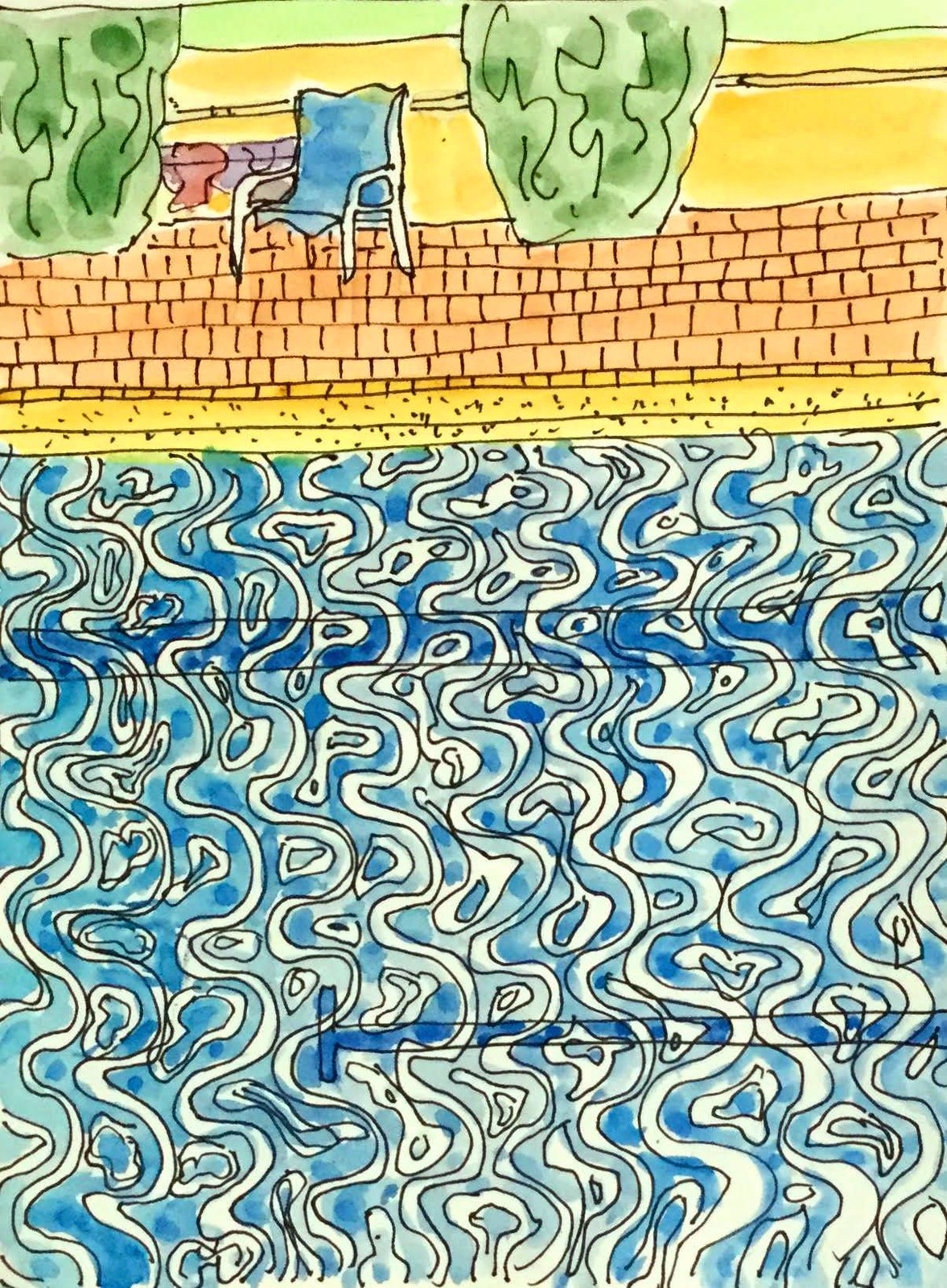This detailed color illustration features a serene swimming pool scene. The pool's water is depicted in a light blue hue, with white shapes artfully drawn on the surface to convey the gentle movement of the water. In the background, a brown-tiled patio or walkway can be seen, stretching across the top of the image.

To the upper left, a lush green tree adds a touch of natural beauty to the scene. A prominent blue lawn chair is placed to the right of the tree, positioned near another verdant green tree. The area directly behind the lawn chair is a continuation of the brown background, possibly indicating more of the tiled patio or pathway.

Notable for its simplicity, the illustration features no text, people, animals, or buildings, focusing solely on the tranquil pool environment and its immediate surroundings.